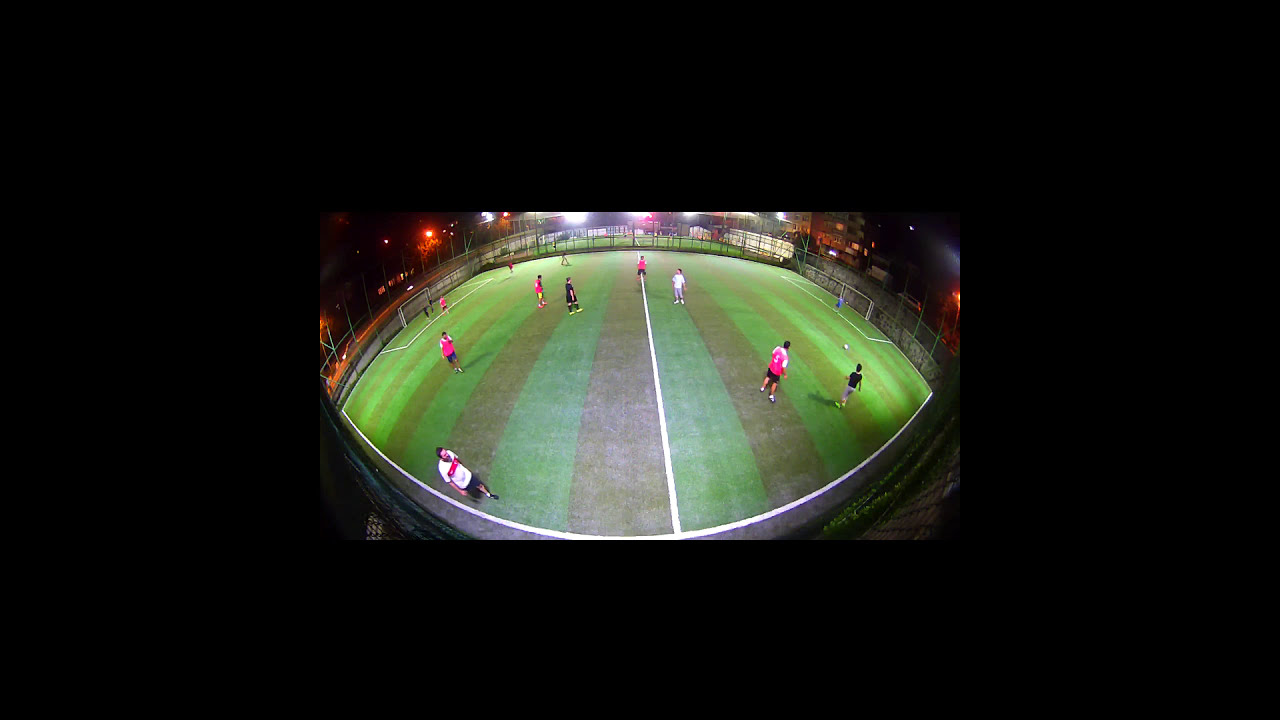This nighttime image, captured from a security camera using a wide-angle lens with a fisheye distortion, shows a soccer field marked by alternating light and dark green stripes. The field is enclosed by fencing, with possibly seating beyond the fence. Bright perimeter lights illuminate the scene, accompanied by warmer yellowish overhead lights. On the pitch, which has the distinctive white lines and goals at each end typical of a soccer field, two teams appear to be practicing. One team wears white shirts with a red stripe and black shorts, while the opposing team is in red shirts with white sleeves. There are eight players and two referees or officials dressed in black. The image suggests a casual practice session, with little action visible and the soccer ball out of sight.